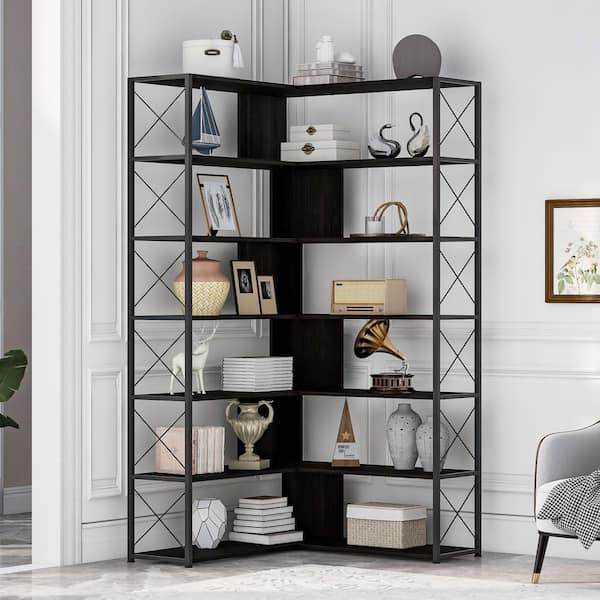The image showcases a sleek, seven-foot-tall, L-shaped black metal shelf designed to fit snugly into the corner of a modern home, against a white wall with crown molding. The shelf comprises six levels, each meticulously adorned with various household items to exemplify its potential uses. The top shelf features a container holding a towel, a stack of books with a white object atop, and a gray circle. The second level displays a ceramic deer sculpture, two storage boxes, and a pair of elegant glass swans. An intricately framed photo and a unique candle occupy the third shelf. The fourth shelf houses a jar, more picture frames, and a model baby vinyl player. Beneath these, a deer sculpture is flanked by stacks of books and a mini gramophone. The bottom shelf contains several books, a trophy, a pyramid, and a stylish vase. Throughout the shelf, you’ll find additional elements like baby swan figurines and a variety of random but organized objects, creating a harmonious and modern aesthetic. Adjacent to the shelf, a chair with some fabric draped over it, a painting, and a potted plant complete the inviting, contemporary scene.